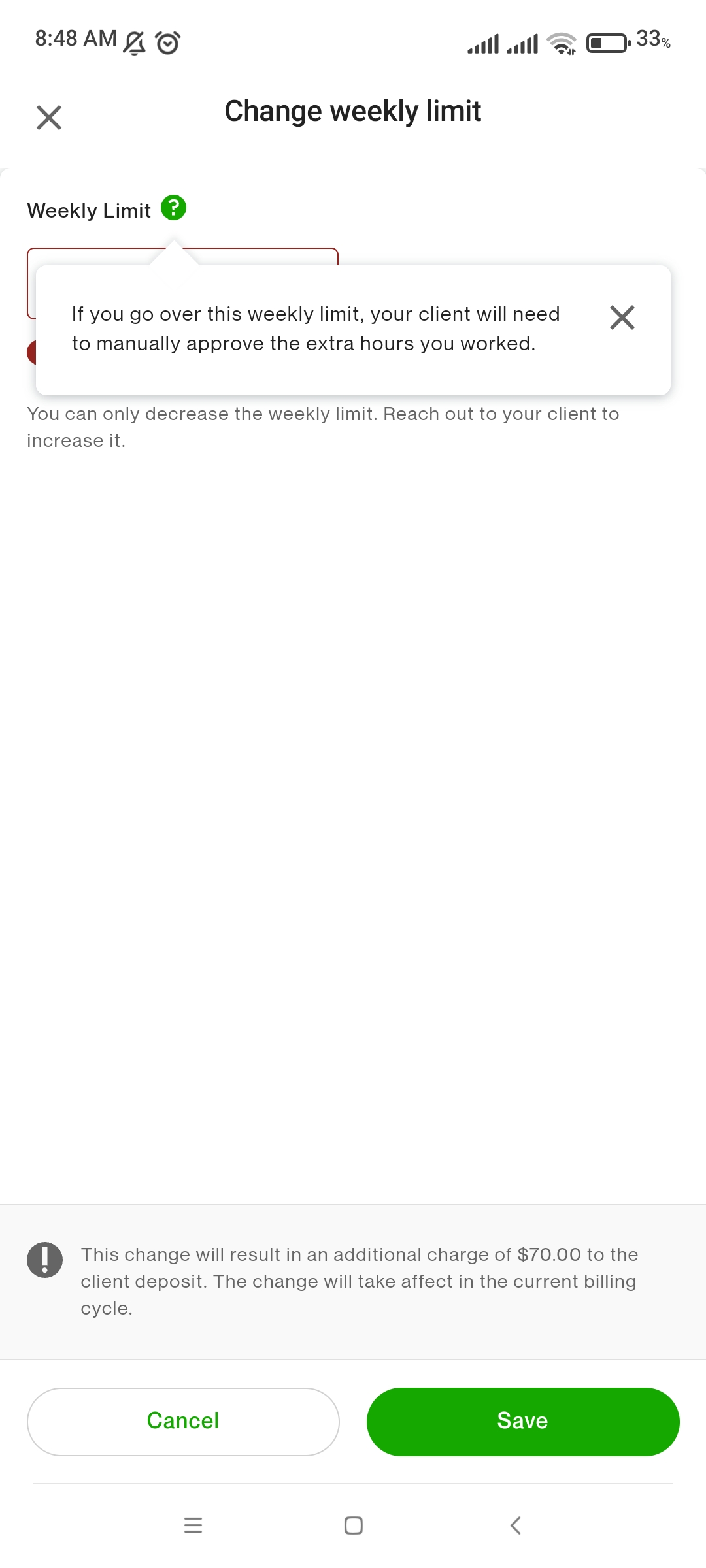A detailed screenshot from a cell phone displays various on-screen elements:

- The status bar at the top indicates it is 8:48 AM, with a muted bell icon, an alarm clock graphic, and status indicators for cellular signal, Wi-Fi connectivity, and battery life at 33%.
- Below the status bar, a pop-up window dominates the screen. It features an 'X' on the upper left corner for closing the window.
- Centrally placed text reading "Change Weekly Limit" followed by another mention of "Weekly Limit" further down.
- A green circular icon with a white question mark is present below these headings.
- Beneath the green circle is a white rectangle containing an informative message: "If you go over this weekly limit, your client will need to manually approve the extra hours you worked." An 'X' is also positioned next to this message.
- The pop-up partially obscures a background element featuring a burgundy-trimmed rectangle with a half-circle design in a burgundy or reddish-burgundy shade beneath it.
- Additional instructional text is visible under the obscured area: "You can only decrease the weekly limit. Reach out to your client to increase it."
- At the bottom of the pop-up, there is a warning section with a light gray background. It contains a circle with an exclamation point and a warning message: "This change will result in an additional charge of $70 to the client deposit. The change will take effect in the current billing cycle."
- Finally, there are two options for the user: 'Cancel' and 'Save'.

This clean, detailed caption captures every critical aspect of the cell phone screenshot, offering an in-depth visual description.